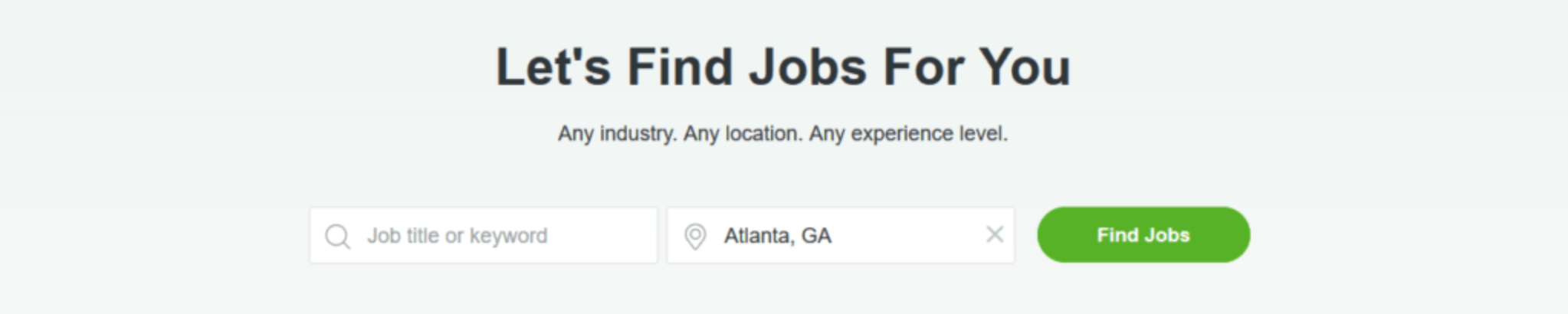In the cropped image of a job-finding website, the main section prominently features the large text "Let's find jobs for you." Just below this headline, smaller text asserts the website's versatility, stating, "Any industry. Any location. Any experience level." The background of the website showcases a very light green to turquoise gradient, lending a calm and inviting feel to the page.

The focused part of the screenshot includes two significant search bars positioned below the textual content. The search bar on the left invites users to input a "job title or keyword" and the placeholder text is displayed in a lighter gray color. In contrast, the search bar on the right is designated for entering a location and currently displays "Atlanta, Georgia" in black text. Next to this location search bar, a location symbol appears on the left, indicating the purpose of the field, with an 'X' on the right to allow users to clear or change the location.

Prominently below these search bars, a green button with bold white text reads "Find Jobs," serving as a call to action for users ready to initiate their job search. The overall layout and elements within this cropped section of the website are designed to make the job search process straightforward and efficient.